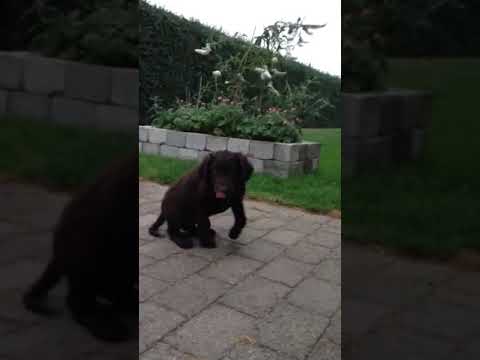This image captures a young black puppy, approximately one to two years old, sitting on a walkway made of gray stone bricks. The puppy appears to be in the process of lifting one of its paws, indicating it's about to get up. The scene is situated outdoors, likely in a backyard or park. Surrounding the puppy is a well-maintained area: to its right, there's green grass and a flower bed bordered with similar gray bricks. This flower bed contains green plants and red flowers, possibly roses or tomatoes, with some weeds growing amidst them. Further in the background, there is a tall, neatly trimmed row of dark green hedges or bushes, which may serve as a fence. Behind the hedges, a green hill is visible, covered with grass or bushes, adding depth to the scene. The sky above is mostly clear with slight overcast, lending a light atmosphere to the setting. The image itself appears cropped, with darkened, zoomed-in borders on the left and right, suggesting it may have been shared on social media platforms like Instagram or Facebook.